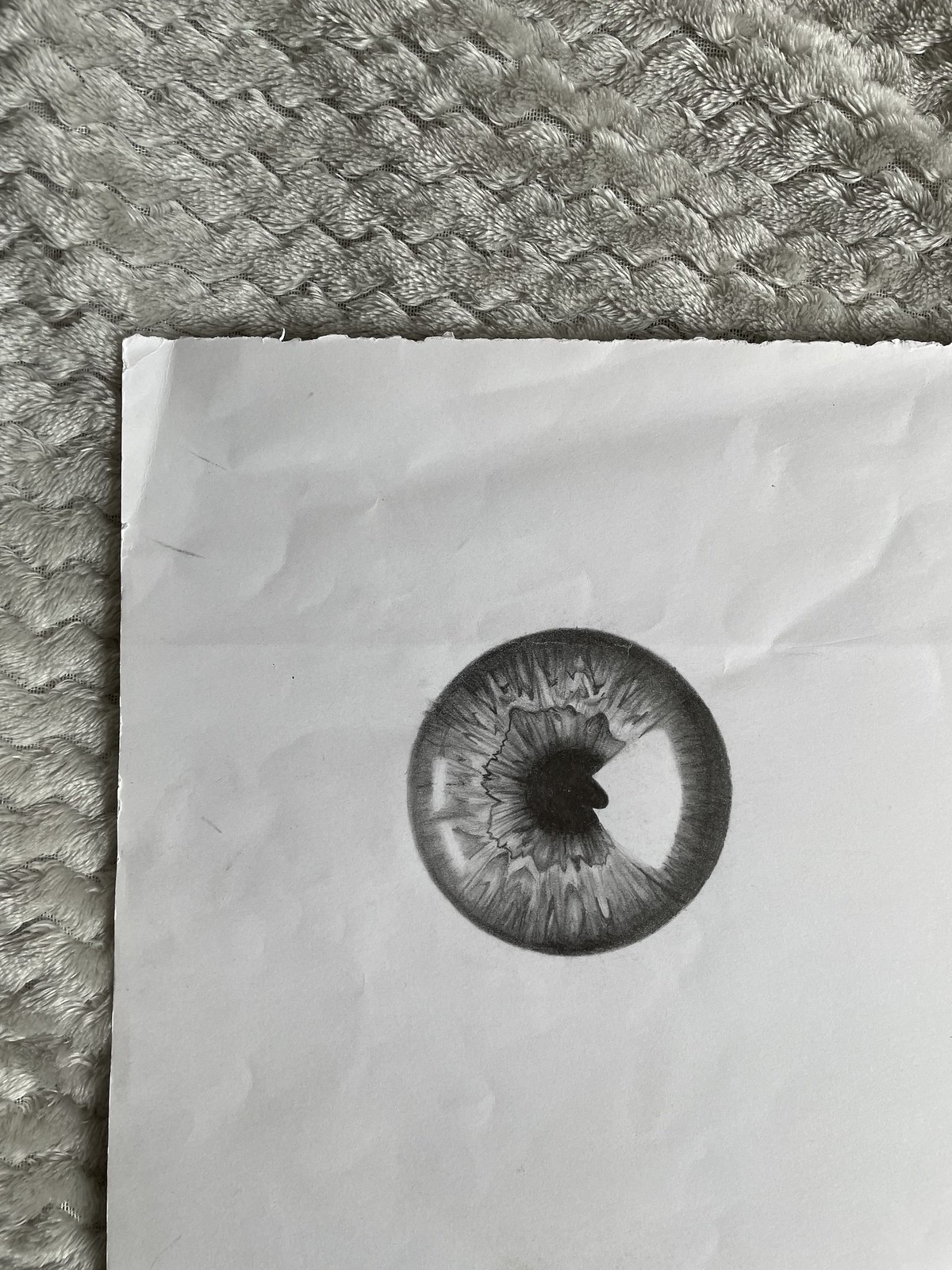The image features a finely detailed pencil drawing of an eye's iris and pupil, rendered on a slightly crumpled white piece of paper that appears to have been torn from a notebook, as indicated by its jagged edges. The piece of paper, roughly positioned in the bottom right corner of the photo, rests on a gray, herringbone-patterned carpet or rug. The drawing itself occupies about 25% of the image and showcases an intricate iris with textured lines converging toward the solid black pupil, which is encircled by a petal-like shape. A striking highlight on the iris suggests a realistic light reflection, enhancing the lifelike quality of the artwork.